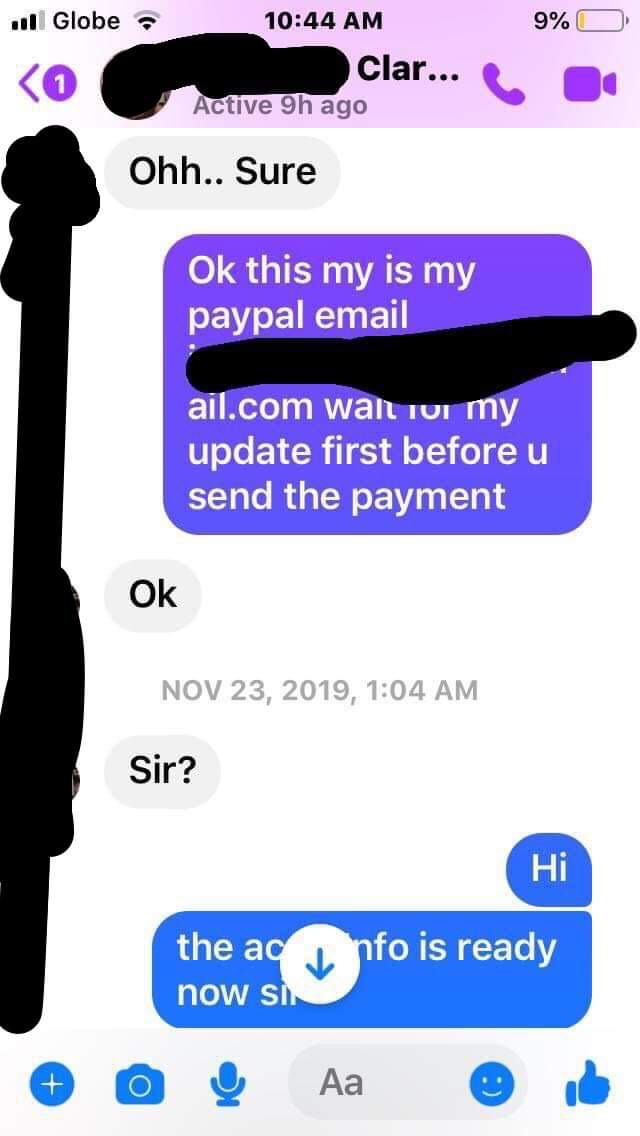This screenshot from a phone depicts a text messaging interface with several pieces of information visible despite some being redacted. At the top of the screen, the status bar indicates it is 10:44 a.m. with a Wi-Fi signal from Globe and a 9% battery life. The header displays a partially obscured contact name, "Claire C L A R...", with icons for a phone call and video call, and notes the contact was active nine hours ago. 

The conversation shows a sequence of messages:
1. "Oh sure..."
2. "Okay, this is my PayPal email [address blacked out]. Wait for my update first before you send the payment."
3. "Okay"
4. A timestamp from November 23rd, 2019 at 1:04 a.m.
5. "Sir?"
6. "Hi, the info is ready now, sir."

The bottom of the interface features action icons including a thumbs up, a blue smiley face for emojis, a microphone for voice recordings, and a camera.